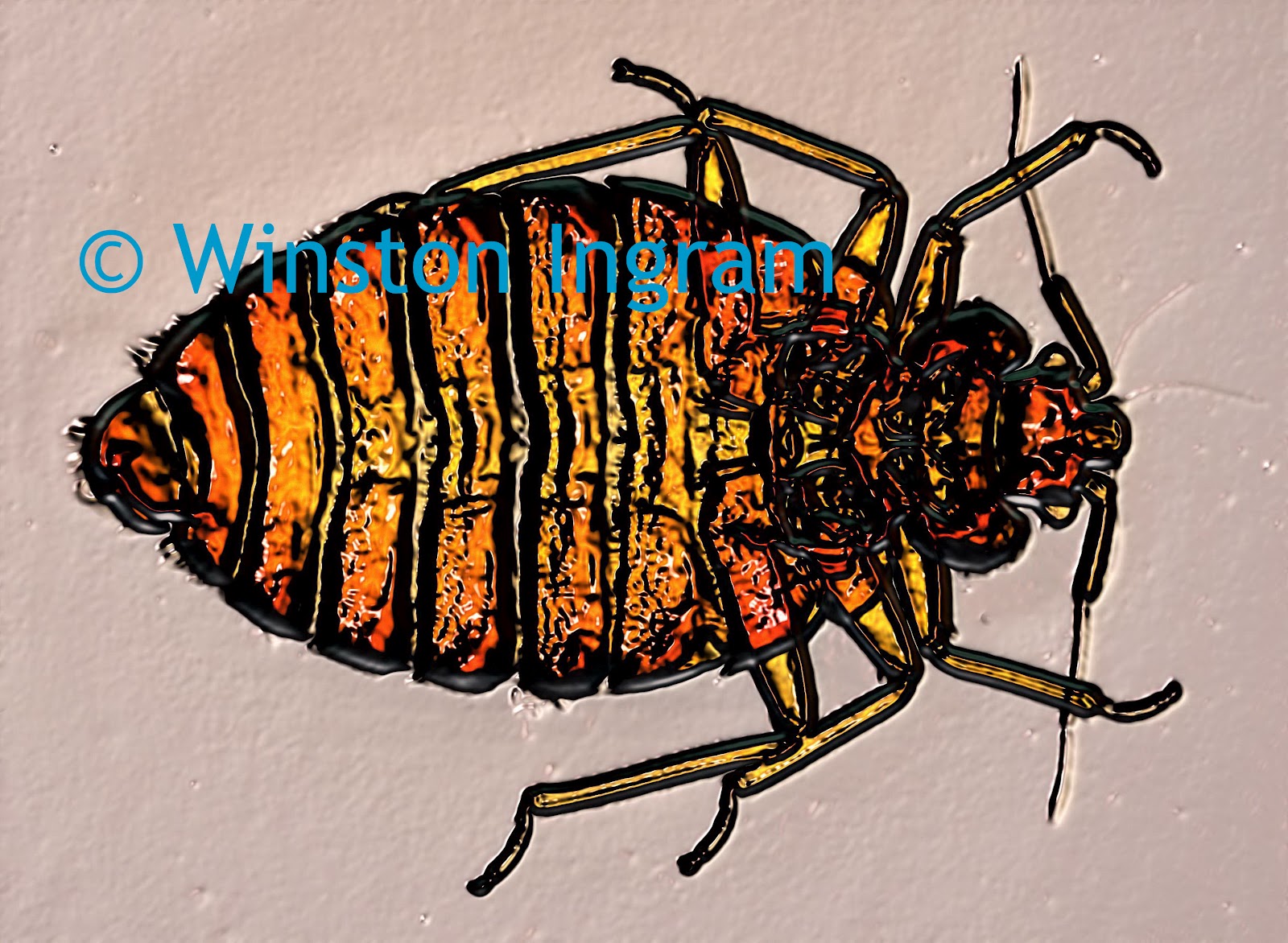This image presents a detailed, microscopic view of a louse, characterized by a distinctive black outline encircling its entire body. The internal body of the louse predominantly showcases orange hues, while its six limbs and antennas exhibit a yellow coloring. The louse's body, including its large striped abdomen, has an intricate pattern resembling tiger stripes with alternating bands of yellowish-orange and black. The small head features two yellow eyes and prominent mouthparts. The image, potentially a manipulated photograph or a highly detailed drawing, appears slightly upside down and is set against a beige backdrop. Superimposed over the louse in blue text is the name “Winston Ingram,” alongside a copyright symbol on its left.